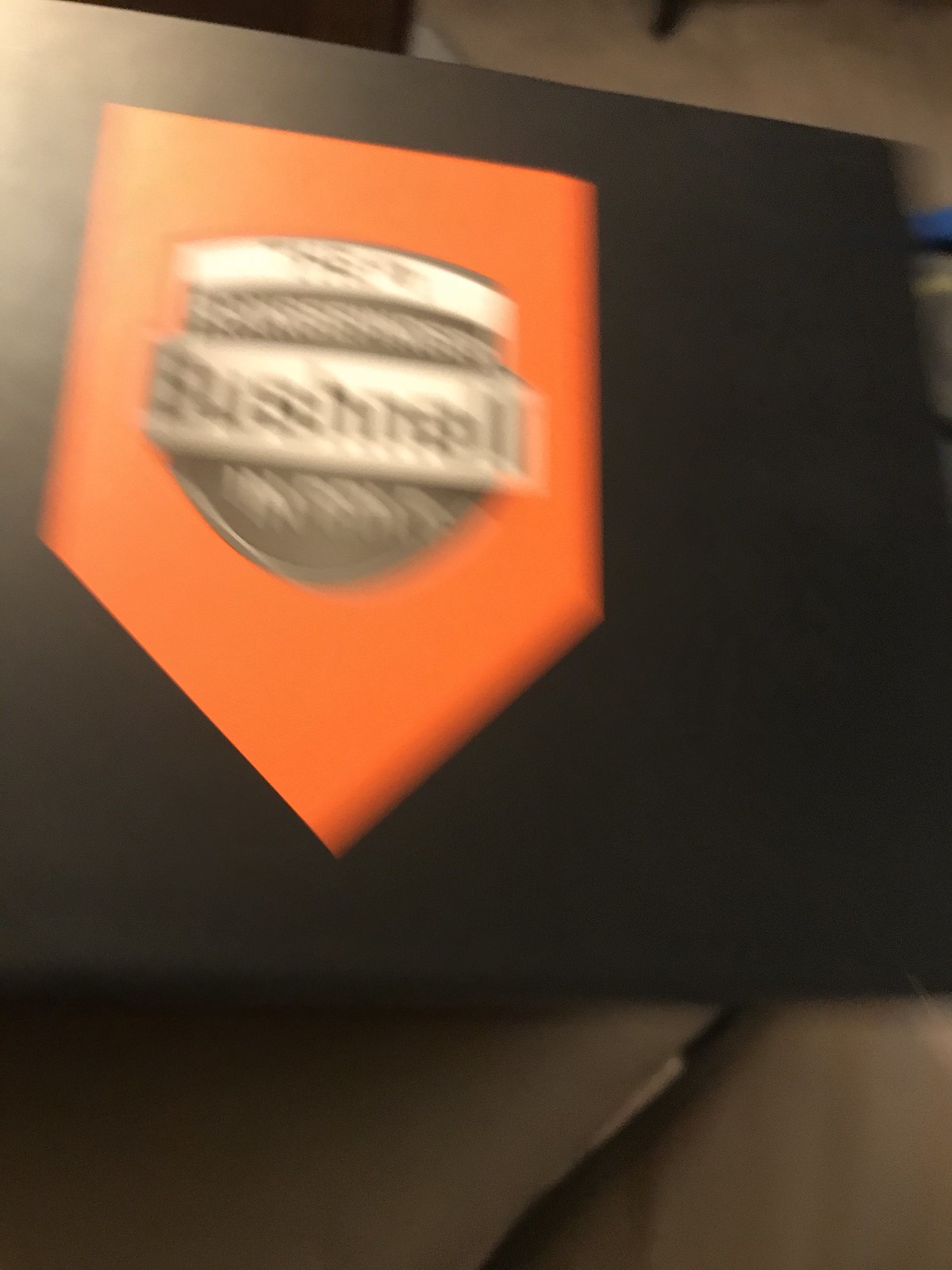In this real-life photograph, we are presented with a top-down view of a black box situated on a beige or khaki-colored surface, which could potentially be a carpet or a floor. The surface is adjacent to a black wire that is partially visible at the bottom of the image. The box's design features a distinct geometric shape resembling an upside-down house: a square base with a triangular top, forming a cohesive singular piece. Within this upside-down house shape is a U-shaped logo accompanied by some text; however, due to the image's blur, the text is not legible. Additionally, there are movement lines around the text and logo, suggesting an attempt to capture a clear image that was unsuccessful. The upper portion of the photograph also reveals more of the khaki-colored background along with hints of dark black or brown elements, which might be parts of furniture such as chair legs.